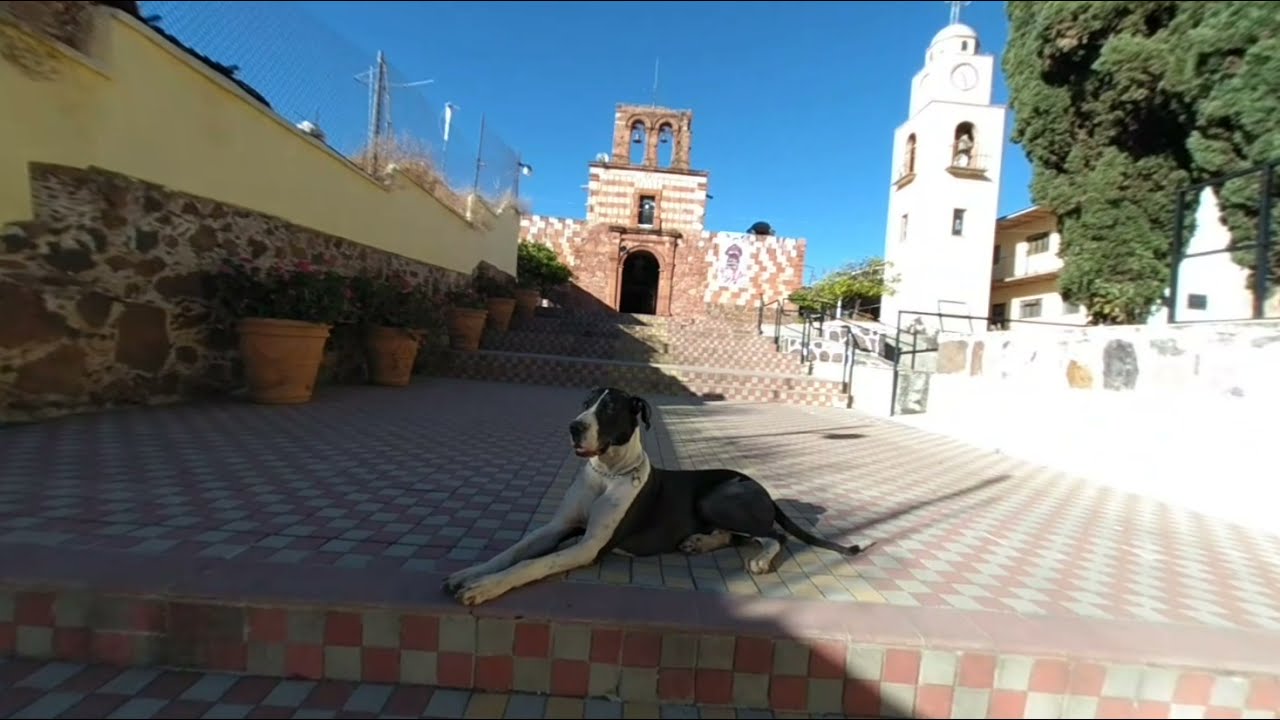In this detailed photograph set in an outdoor environment, a large black and white dog lies sprawled out on checkered tile steps of red and cream hues, positioned centrally towards the bottom of the image. The steps themselves are shallow and flat, leading up to a larger tile building. Ascending on the left side of the steps, large tan clay pots filled with lush plants form a vibrant row. On the right side, intricate black stair railings complement the lighter colored tiles. In the distance on the right, there is a narrow white clock tower extending upwards, flanked by additional buildings and greenery, visible in the top right-hand corner. The composition, devoid of any text, captures a tranquil city square scene, rich in architectural and natural elements.